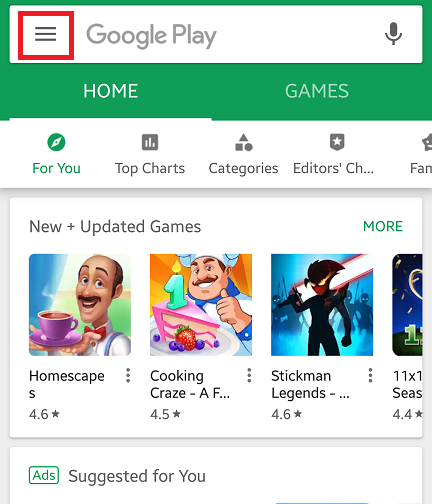A screenshot of the Google Play Store interface. At the top, there's a green header with a white banner inside that displays "Google Play" in prominent text. Below that, there are navigation options with "Home" in white text on the left and "Games" on the right. Proceeding downward, there's a segmented bar featuring different categories or topics. The top categories include "For You" highlighted in green with green text and icon, followed by "Top Charts," "Categories," and "Editor's Choice" in gray text with corresponding gray icons.

Beneath these segments, there is a white rectangular section titled "New and Updated Games" in gray text on the left, with the word "More" in green text to the right, indicating additional content is available. This section showcases various game suggestions such as "Homescapes," "Cooking Craze," and "Stickman Legends," each accompanied by an illustrative image. 

"Homescapes" features an animated image of a man holding a cup of coffee. "Cooking Craze" displays a chef presenting a birthday cake with a green one-year birthday candle. "Stickman Legends" shows a character in black set against a blue background with silhouetted soldiers in the backdrop. The visual representation of each game provides a glimpse into their themes and aesthetics.